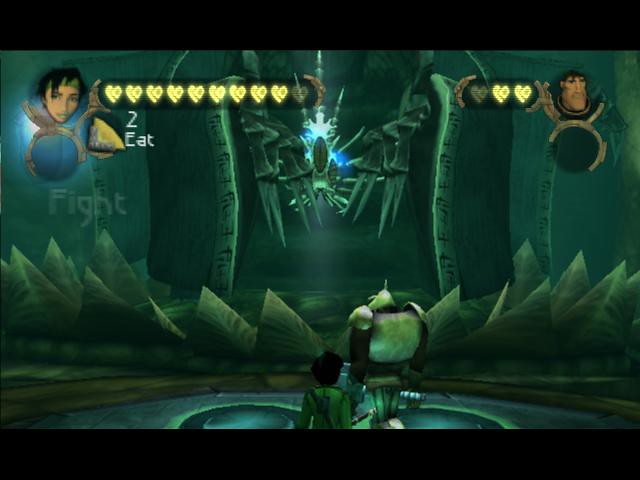The image is a screenshot of a futuristic video game scene dominated by shades of green. In the top corners, there are two cartoon-style character faces, likely representing players on different teams. The left-hand character has 10 out of 11 yellow hearts, while the right-hand character has 2 out of 3 yellow hearts, indicating their remaining lives. Beneath the left-side hearts, there is the number "2" and the word "EAT," along with an icon of a food item.

The background features a dark green hue, adorned with pointed shapes resembling leaves or spikes opening like petals. These spikes encircle a central structure, reminiscent of a Star Trek-like portal with blue lasers illuminating stylized thorns and posts inscribed with hieroglyphics.

In the foreground, a human figure in armor stands with their back to the viewer, accompanied by a shorter figure with dark hair, who appears to be a robotic companion. They face a creature in the center that looks like a spider with illuminated tops. The scene is framed by plain black bands at the top and bottom, completing the screenshot’s aesthetic.